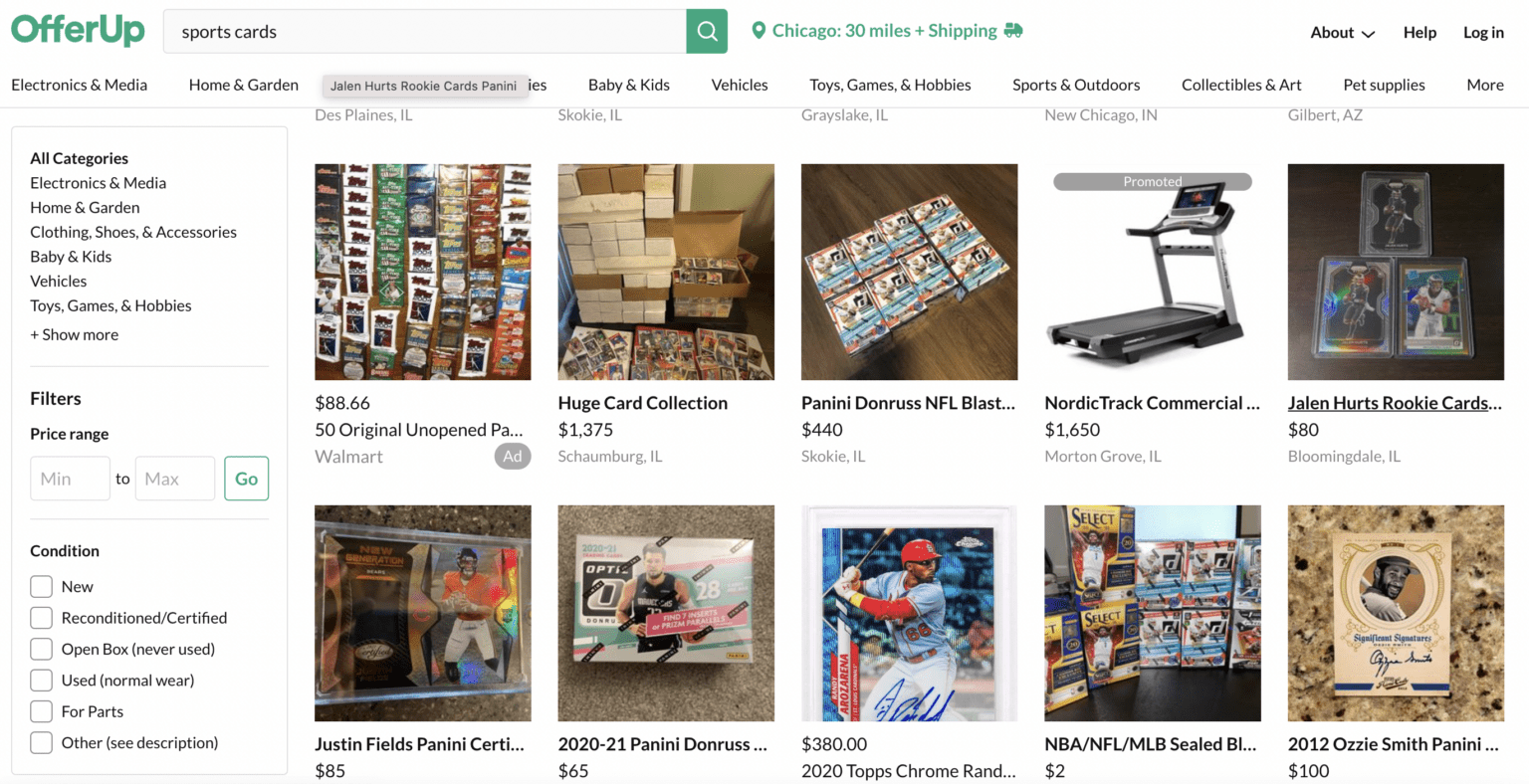In this image of OfferUp, a popular online marketplace, the browser search bar has been populated with the term "sports cards." A green search icon is prominently displayed beside the search input field which specifies a 30-mile radius around Chicago for the search with shipping enabled. The results display a variety of images depicting items available for purchase, predominantly focusing on sports trading cards. Despite the focus on trading cards, a NordicTrack commercial machine also appears amidst the search results. The photographs of sports cards vary; some show multiple cards grouped together, some offer close-up shots, and others present singular cards, although some images lack clarity and detail making them hard to see.

On the left-hand side of the screen, there is a sidebar labeled "All Categories," listing various product categories such as electronics and media, and vehicles, among others. In the center, the screen shows options for applying filters, including selections for price range. At the bottom section of the interface, the condition of items can be filtered with options like new, used, reconditioned, for parts, and others with descriptions. The top menu bar includes navigational options like Help, Login, and an About section with a drop-down menu. The categories are also listed horizontally across the top of the screen for easy accessibility.